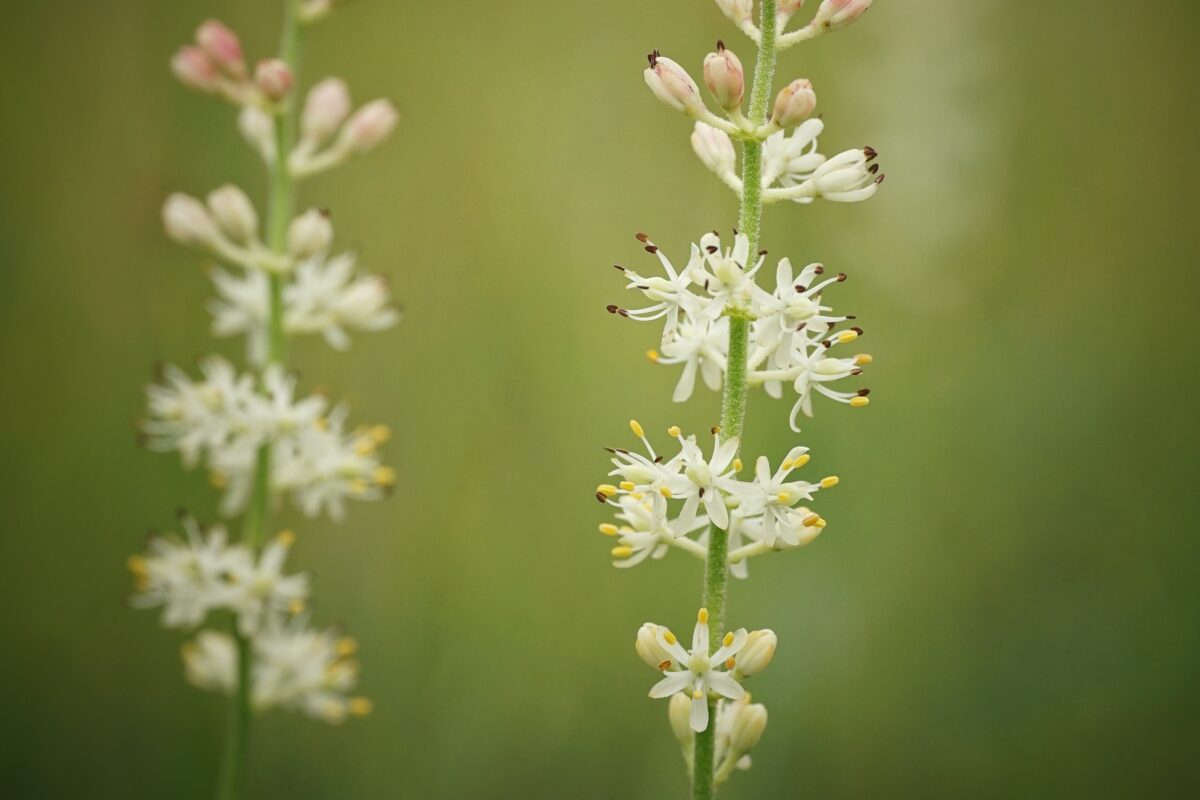In the image, there are two prominent plants of the same species, each featuring multiple small, delicate flowers with six petals. The plant on the right has a green stem that appears thick and possibly velvety, with clusters of flowers spaced about an inch to an inch and a half apart. The flowers are predominantly white with some showing yellow or brown tips, and a few are still in bud form, waiting to bloom. Similarly, the plant on the left mirrors this structure but is not in focus. The background is a blurred mix of green hues, enhancing the focus on the intricate details of the flowers and stems in the foreground.